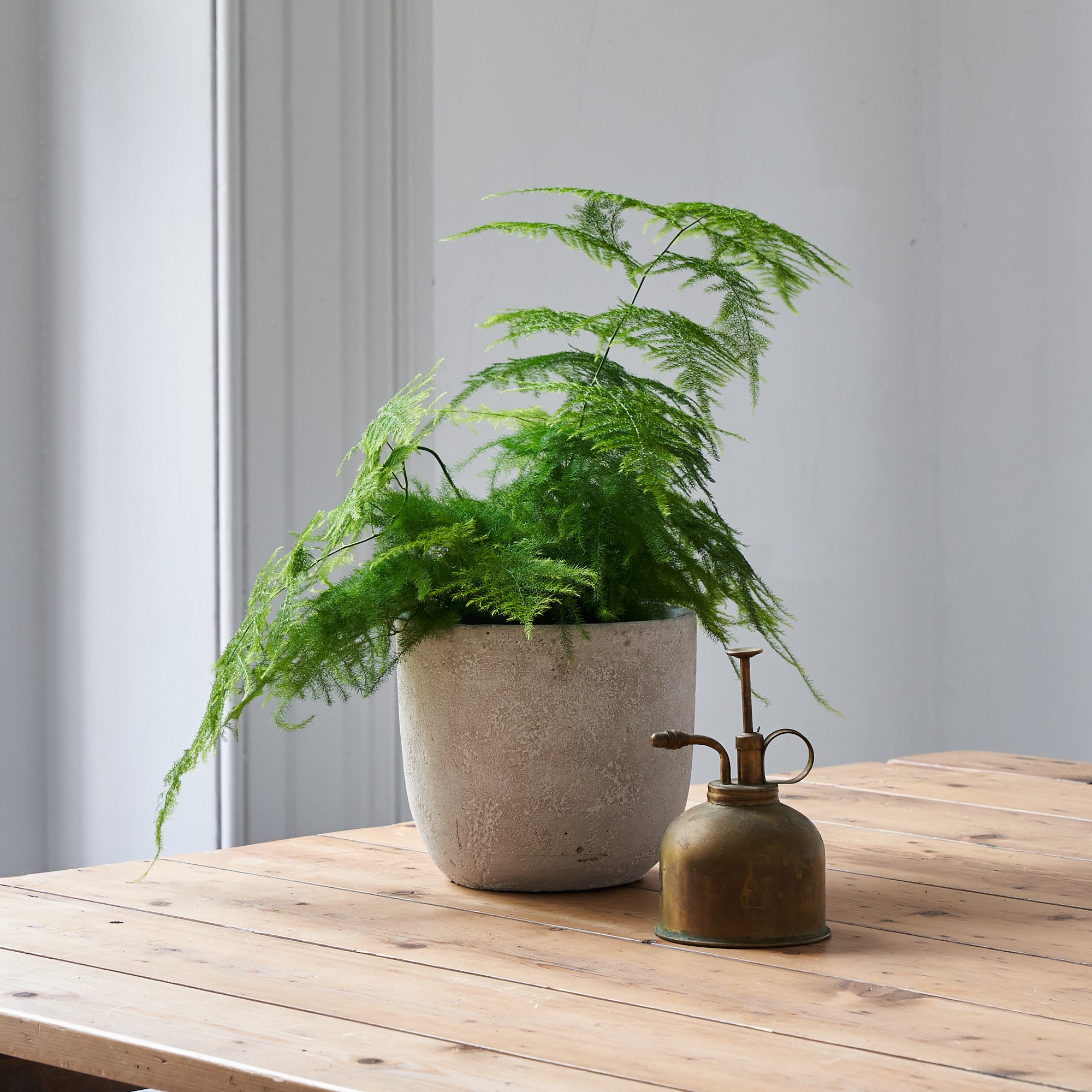In this image, we see a potted plant with vibrant, fuzzy green foliage, exhibiting a slightly wild and untamed growth pattern. One of its stems extends to the right, while another part cascades toward the bottom left. The plant, which resembles a fern, is housed in a weathered, grey stone or cement pot that sits atop a rustic, light brown wooden table made of visible planks. To the right of the plant is a vintage metal sprayer, possibly made of copper or brass, featuring a curved spout, a looped handle at the back, and a pump mechanism on the top for dispensing liquid. The background is a simple white room, providing a clean and unobtrusive backdrop for the scene.